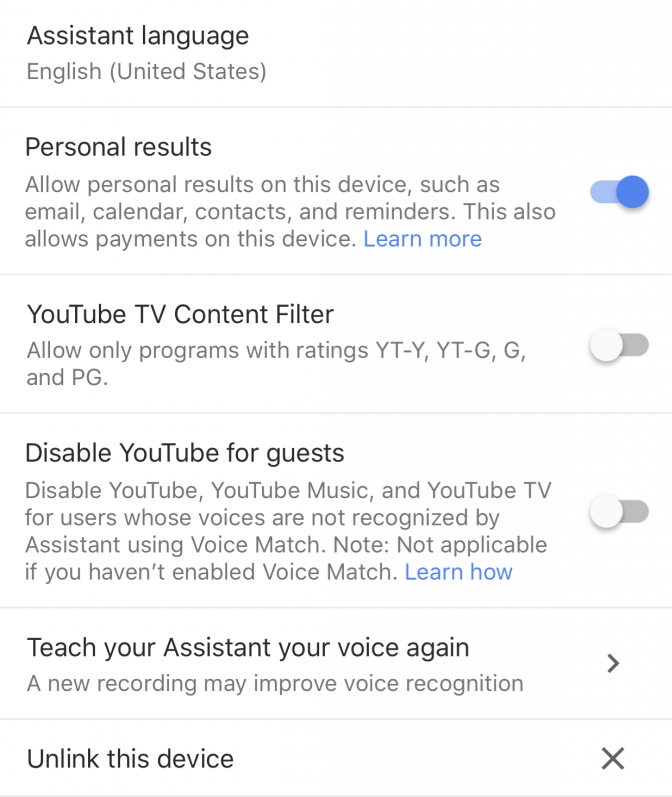The image features a settings interface on a white background. At the top, in black text, it reads "Assistant Language". Below that, in gray text, it indicates "English (United States)". 

A horizontal line spans the width of the image, demarcating the section that follows. Beneath this line, the phrase "Personal Results" is displayed in black text. Directly underneath, in gray text, there is an explanation reading, "Allow personal results on the device such as email, calendar, contacts, and reminders. This also allows payments on the device." 

Further down, a blue hyperlink labeled "Learn More" is positioned above a blue toggle switch, which is set to the "on" position, signifying that personal results are enabled.

The next section reads "YouTube TV Content Filter" in black text. In gray text below, it states, "Allow only programs with ratings YT-Y, YT-G, G, and PG." Adjacent to this description is a gray toggle switch, which is in the "off" position.

The final section of the interface mentions "Disable YouTube for Guests" in black text. The accompanying gray text provides additional details: "Disable YouTube, YouTube Music, and YouTube TV for users whose voices are not recognized by Assistant using Voice Match. Note: not applicable if you have enabled Voice Match."